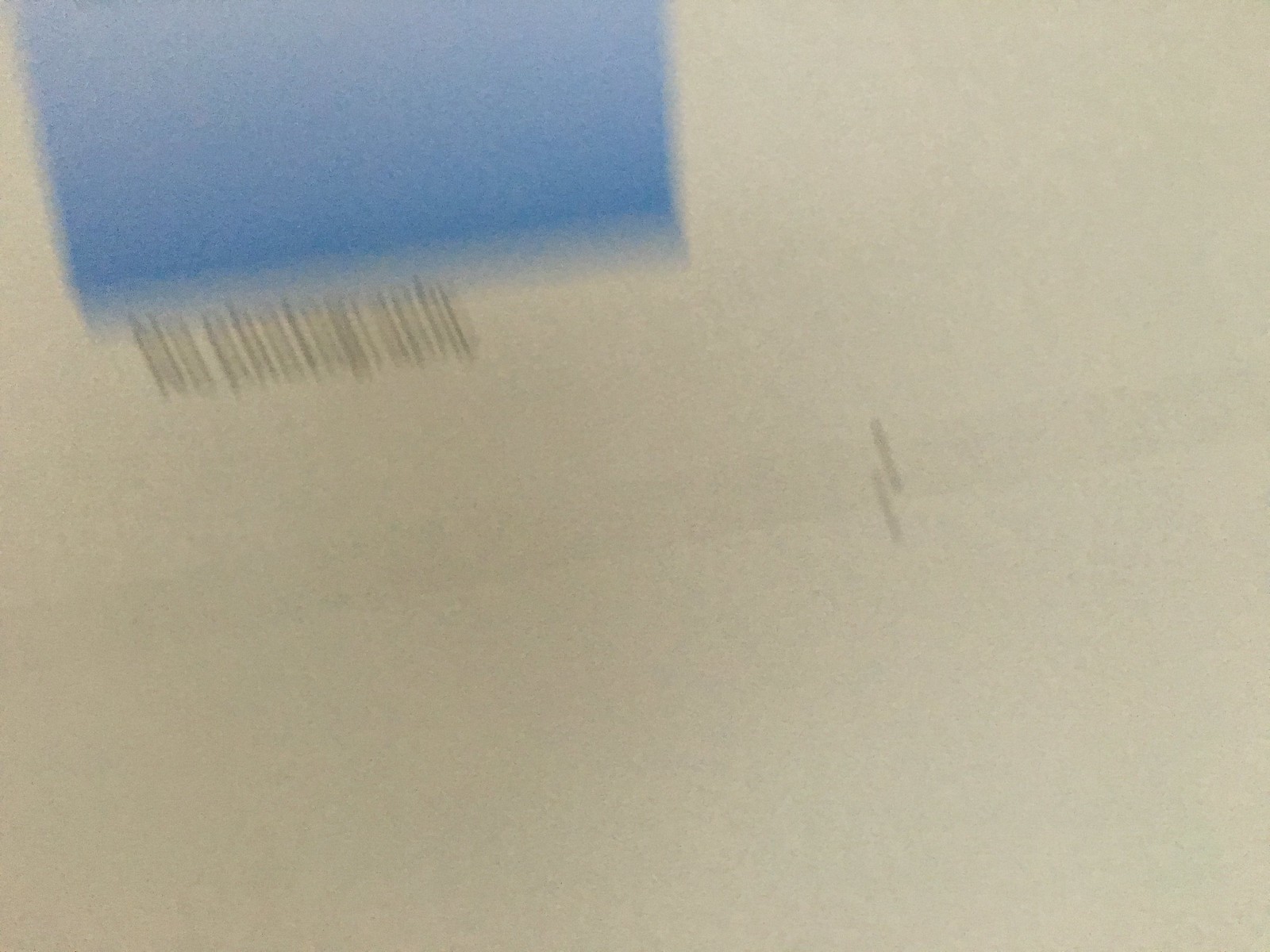The image depicts an extremely blurry photograph of a white piece of paper that appears to have some text written on it. The text includes "No Photography" written in black letters, though the blurriness significantly obscures the clarity. Above this text, there is an indistinct blue blur suggesting perhaps a header or logo. The paper also features two black lines in the center, though they too are blurred and lacking definition. The background of the image is predominantly white, contributing to the overall indistinctness of the photograph.